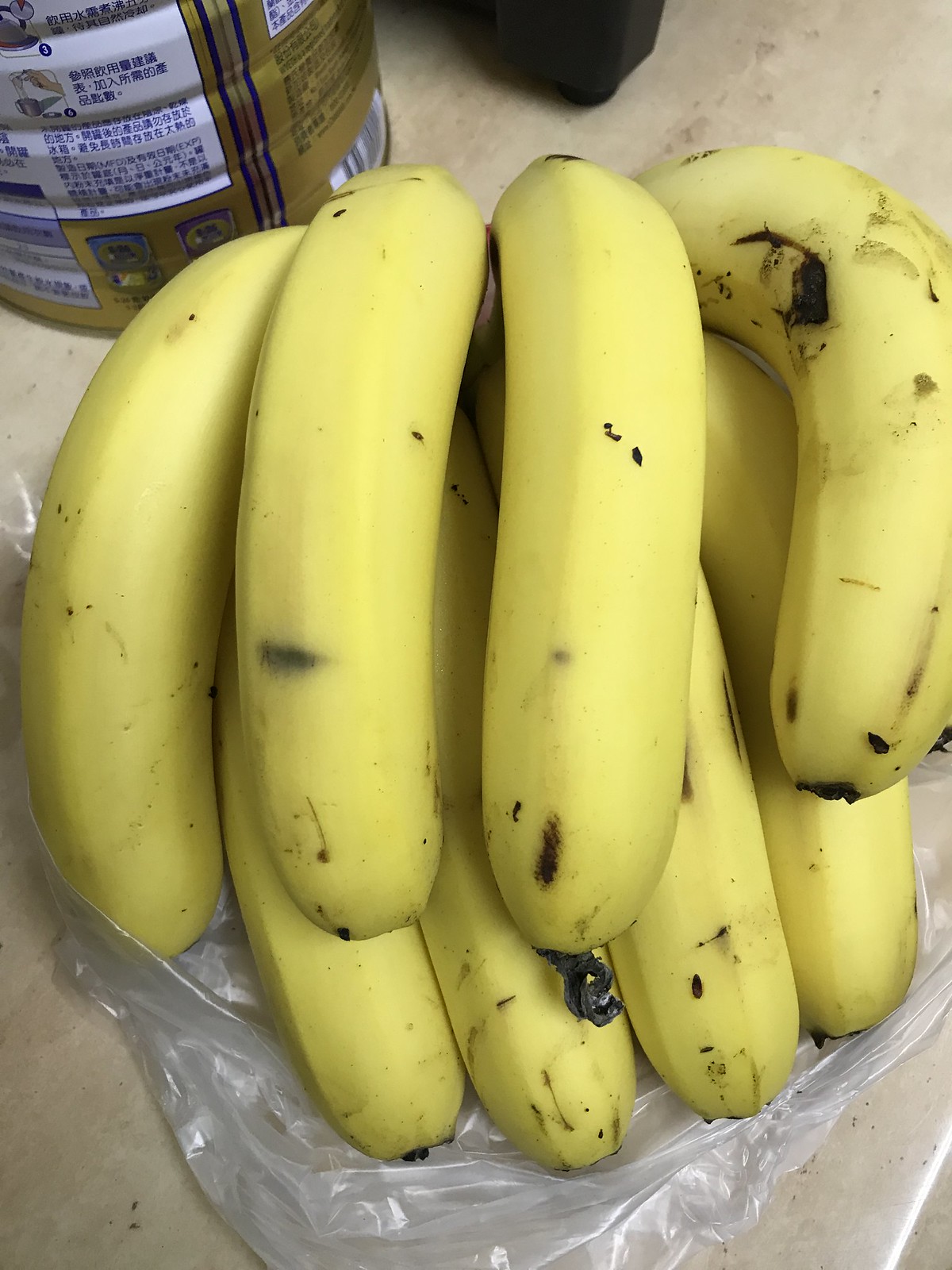This photograph features a bunch of eight ripe, yellow bananas with some brown bruising, arranged vertically with their stems pointing downward and backsides facing up. The bananas are partially enclosed in a clear plastic bag, likely the one they were purchased in, which rests on a light-colored stone countertop resembling marble but not quite it. The countertop features subtle markings, adding texture to the surface. In the top left corner of the image, there is a golden coffee can with blue stripes, white label sections, and Asian characters, likely in Chinese or Japanese. The can also displays an image of a hand pouring something into a cup. The overall focus of the image is the bananas, which dominate the frame, lying longitudinally in two layers of four.